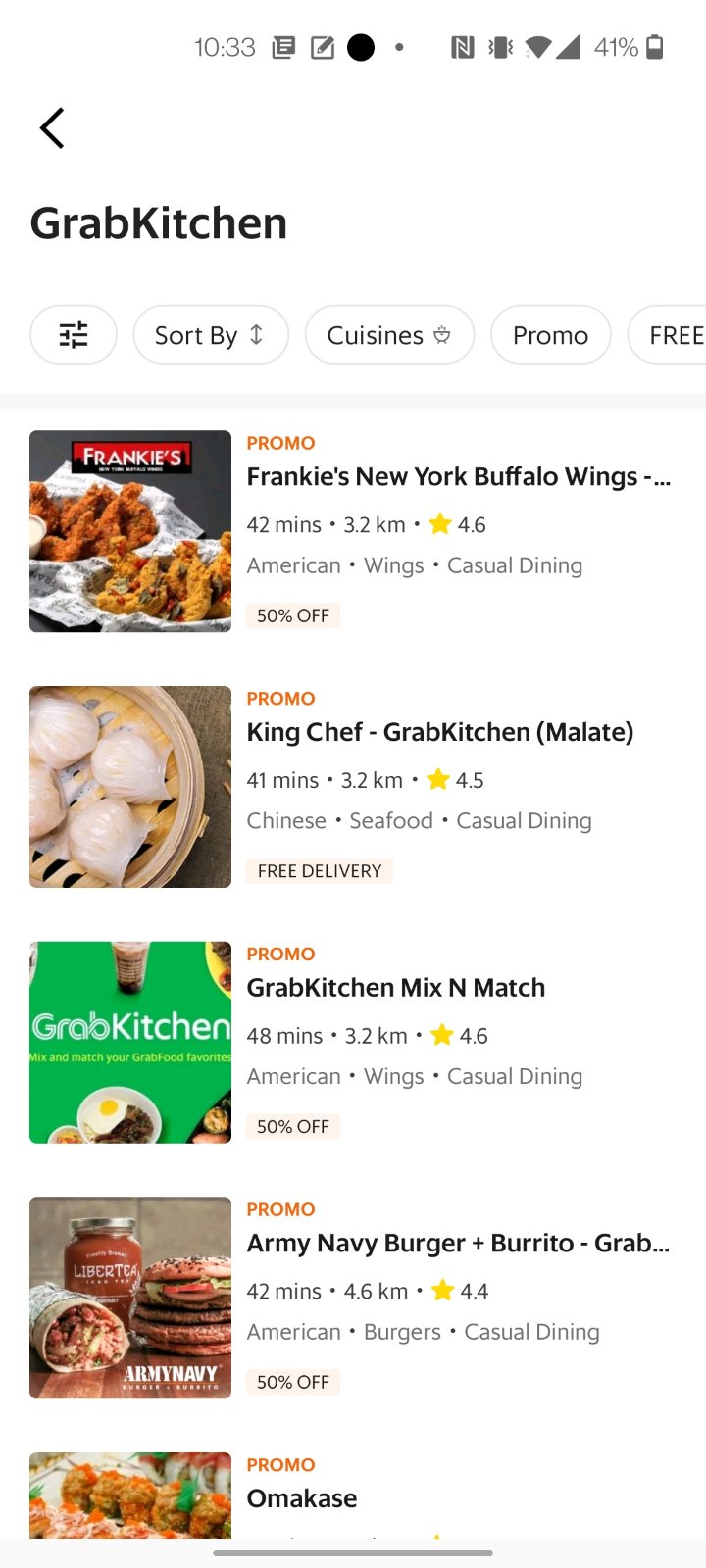In the image, a phone screenshot is displayed. Starting from the top right corner, there is a battery icon indicating 41% charge remaining. To the left, the signal strength and Wi-Fi icons are both fully filled, signaling strong connections. A phone vibration icon is also present. On the top left, the current time is shown as 10:33. Just below the time, a black-colored back arrow is positioned on the far top left, and beneath it, the bold black text reads "Grab Kitchen."

Underneath the "Grab Kitchen" title, there are several category options: a filter icon, "Sort by", "Cuisines", "Promo", and "Free." The main content of the screenshot features a list of five restaurants:

1. **Frankie's New York Buffalo Wings**: 42 minutes away, 3.2 kilometers, rated 4.6 stars.
2. **King Chef Grab Kitchen Malate**: 41 minutes away, 3.2 kilometers, rated 4.5 stars.
3. **Grab Kitchen Mix and Match**: 48 minutes away, 3.2 kilometers, rated 4.6 stars.
4. **Army Navy Burger**: [partial data]
5. **Omakase**: [partial data]

The screenshot provides a concise overview of the Grab Kitchen interface, detailing the various restaurant options and their respective distances, delivery times, and ratings.